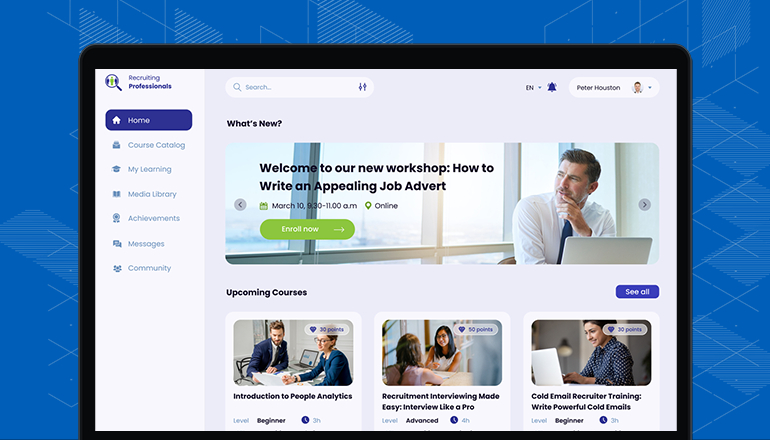The image is a detailed screenshot of a laptop displaying the "Recruiting Professionals" website. The laptop screen's plastic frame is visible, emphasizing the authentic appearance of a device being used. On the upper left-hand side of the website, there is a vertical menu. The menu includes several options listed in the following order: Home, Course Catalog, My Learning, Media Library, Achievements, Messages, and Community.

In the center top section of the screen is a prominent photograph featuring a man in a tie, facing the camera. He is seated in front of a laptop, with what seems to be an office window in the background, indicating he is in a professional, indoor office space. The photograph is captioned, "Welcome to our new workshop: How to Write an Compelling Job Advert."

Additionally, on the website, there is a section labeled "What’s New?" positioned to provide updates or news, although no further details are provided about its content.